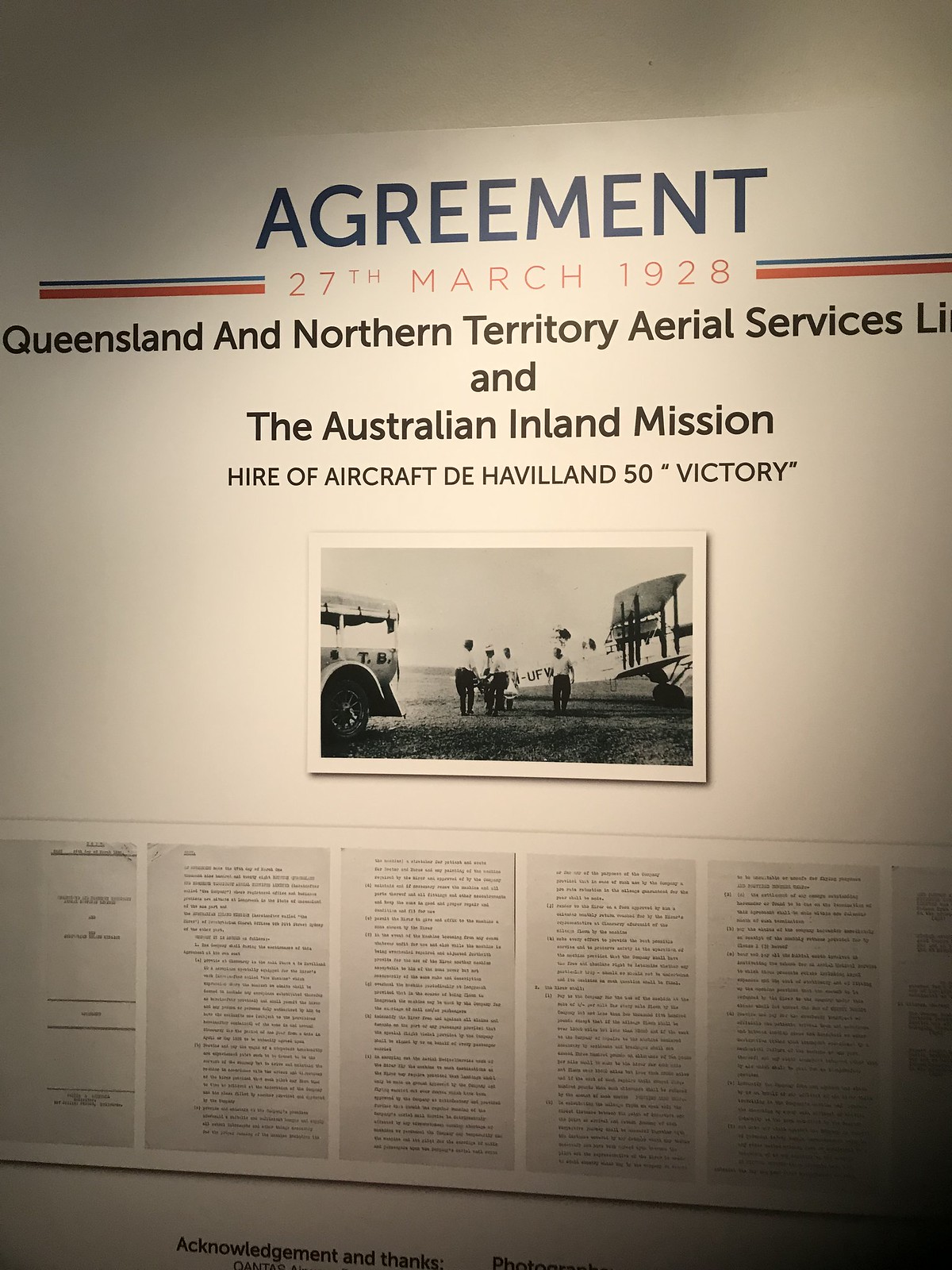The image depicts an informational sign spanning much of a white-painted wall, most likely found in a museum. The wall features multiple lines of text and a centrally placed black and white photograph. At the very top of the sign, in blue font, it reads "Agreement," followed by "27th March 1928" in red font. On either side of the date are thick red bars with thin blue bars above them. Below the date, in three lines of black text, it reads "Queensland and Northern Territory Aerial Services LI" and "The Australian Inland Mission." A smaller black text line underneath states, "(Hire of Aircraft D Haveland 50 Victory)." The black and white photograph shows multiple people standing next to an old-fashioned biplane, with a partially visible car on the left side. Below the photograph, there are six pieces of paper with illegible text. The overall style suggests a historical or commemorative display, focused on an aviation agreement involving the Australian Inland Mission.